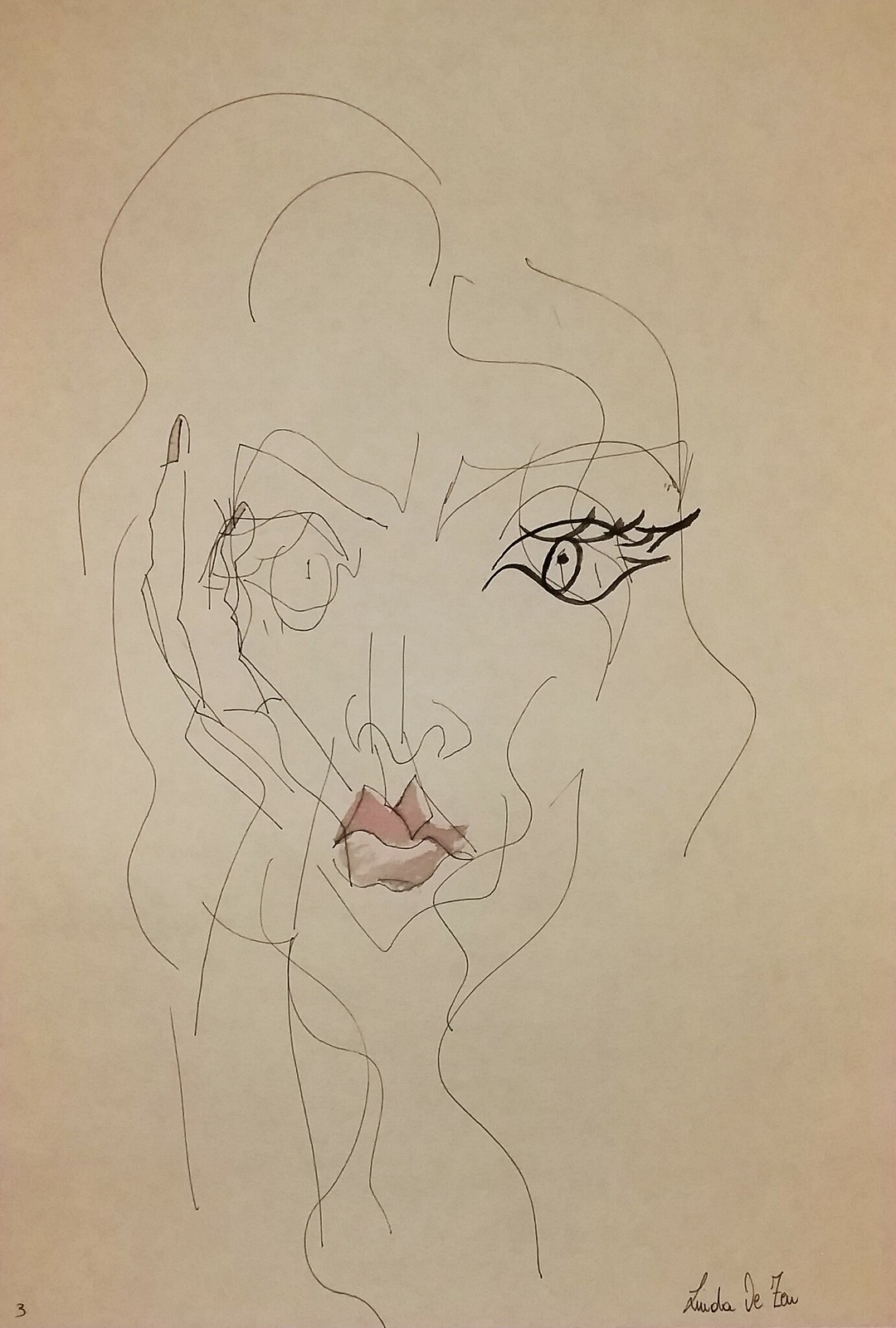The image features an off-white sheet of paper, with a subtle reddish gradient along the edges that might be due to the lighting. The primary subject is a sketch of a woman's face, executed with very fine lines, suggesting the use of a pencil or fine pen. The face includes delicate hair strands framing it and extends to a narrowly drawn neck. Notably, the eyes are asymmetrical; the left eye is detailed with a black marker, giving it depth, while the right eye is simpler, just a circle, likely drawn with the fine pen. The lips exhibit nuanced shading in pink and brown hues, and there's a small brown shading visible on one of the fingernails. At the bottom of the page is a signature in small cursive writing, partially legible. The first name appears to be "Linda," while the last name seems to start with "De," followed by a "Z" and possibly ending with "A-U."